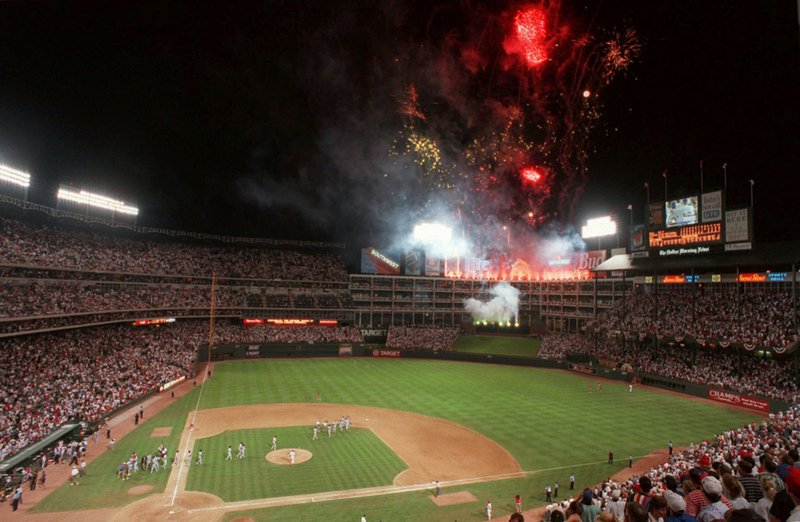The photograph captures a vibrant nighttime scene at Choctaw Stadium in northwest Arkansas, viewed from an elevated vantage point. The stadium, filled with enthusiastic fans, is bathed in artificial stadium lights that illuminate the intricate crisscrossed green grass of the playing field. The infield, showcasing a diamond shape towards the bottom left, features white lines and bases with a green square at its center and a brown circle marking the pitcher's mound. A line of baseball players in gray uniforms walks from the left side of the field, possibly indicating the end of the game. In the top right corner, dazzling red and yellow fireworks explode against the black sky, leaving trails of smoke from the launchers. The home plate is positioned at the bottom left of the image, with the first base located centrally at the bottom, completing the picturesque and dynamic landscape of the stadium.